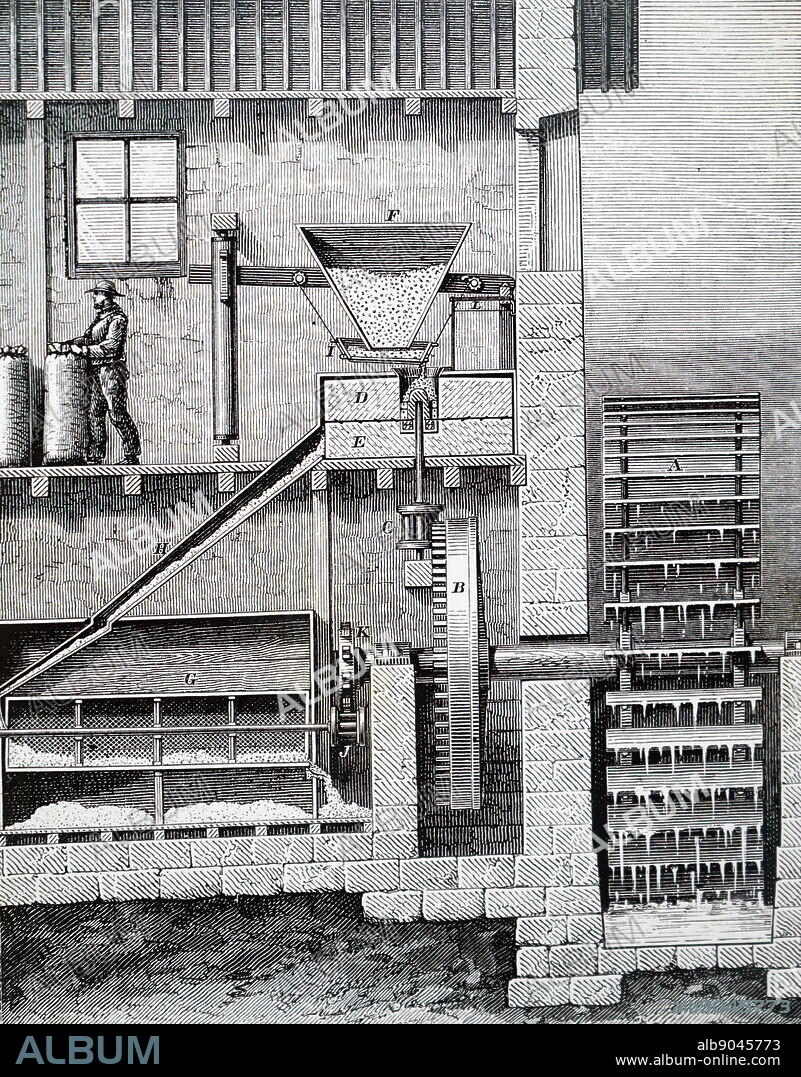This black-and-white illustration depicts the intricate function of a water wheel within a grain mill. To the top left, a man stands by, his hand resting on a large sack that reaches above his waist, seemingly filled with grain. Dominating the right side and bottom of the image is the water wheel, marked 'A,' its wooden slats detailed with vertical and horizontal lines, actively dripping water from an unseen river's flow. Attached to the wheel is a pivotal post, which in turn connects to a large internal cogwheel labeled 'B.' This cogwheel meshes with another, marked 'K,' above it, initiating a sequence that includes an additional cog labeled 'J.' 

To the left of these gears lies a container marked 'G,' where grain or similar material descends. Above this assembly, at the very top, sits a funnel-shaped apparatus labeled 'F,' directing its contents into areas marked 'D' and 'E' for grinding or further processing. This system efficiently transfers the ground substance down into the 'G' receptacle below. The entire mechanism is part of a building, possibly a mill or farm, highlighted with watermarks indicating its copyrighted status (ALB 9045773, www.album-online.com), and a watermark reading "album" scattered throughout the image.